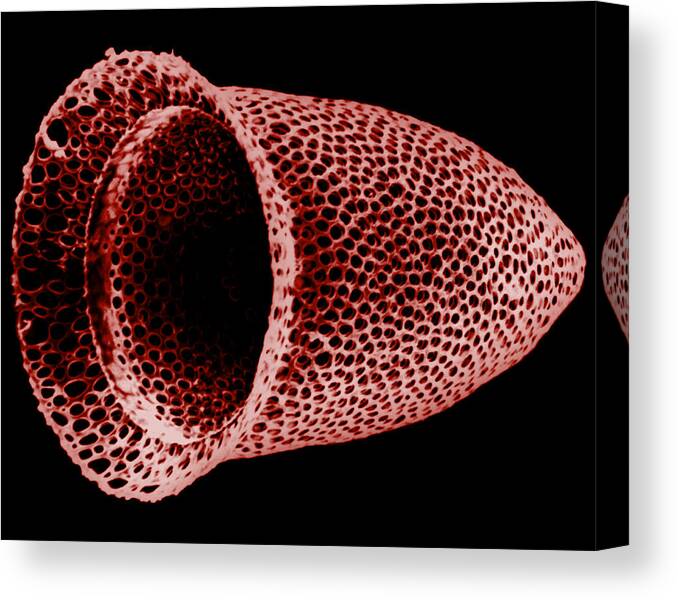The image depicts a highly magnified, scientifically-oriented photograph of a ciliate protozoan, presented in a landscape orientation on a solid black background. The organism features a distinctive, conical or thimble-shaped body that tapers to a point on the right side, with a wide, flared opening on the left. The surface exhibits a lacy structure with an array of irregularly sized, dark spots or holes, transitioning from a reddish-pink to a bronzed hue. The conical shape creates an impression of depth with its shadowed or black center, adding a visually compelling contrast. The entire image has an artistic quality, resembling a detailed, organic form stretched across the canvas, showing intricate biological textures and patterns.